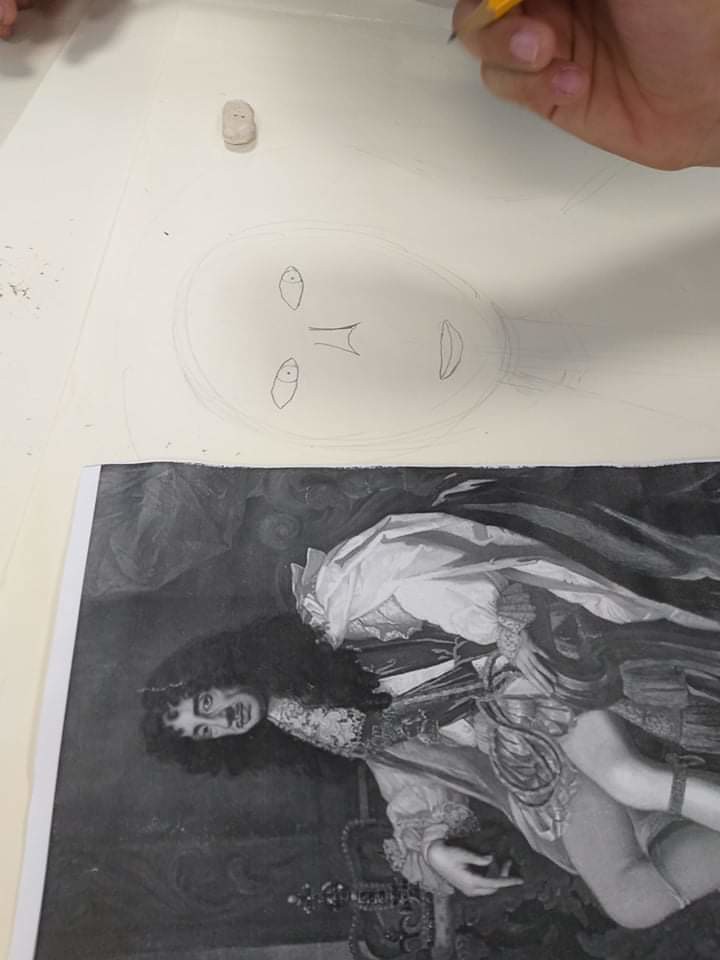This detailed scene captures an indoor color photograph rotated 90 degrees to the left, merging history and art in a unique perspective. The bottom section of the image showcases a regal black and white sketch depicting a Duke or Earl, possibly from the early to mid-1800s. Seated aristocratically, the figure boasts long, curly black hair and is adorned in traditional Victorian attire complete with stockings and a ruffled collar. He rests his right arm on an ornate table beside a crown, hinting at his royal status.

In stark contrast, the upper half of the photograph features a blank expanse of white drawing paper where an amateurish attempt to replicate the noble's portrait is in progress. The nascent sketch comprises a large, simplistic oval face, almond-shaped eyes, a rudimentary nose, and childishly drawn lips. A portion of a right hand, gripping a pencil, is visible in the upper right corner, adding life to the scene. A small white eraser lies near the top edge, left of center, ready to correct any mistakes.

The photograph, devoid of any text or print, compellingly juxtaposes the crude beginnings of an artist's effort against the refined elegance of the historical figure, offering a poignant commentary on the intersection of art and history.